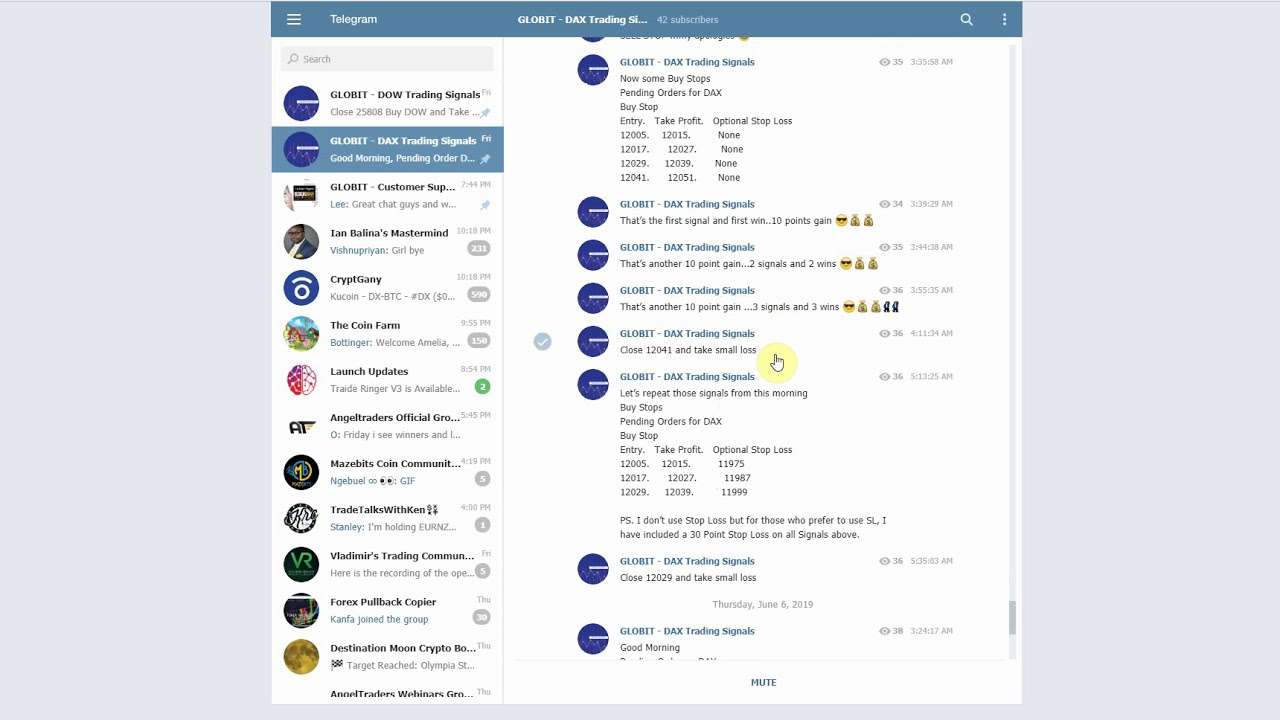This image, sourced from a website, features a meticulously detailed design with a clean and structured layout. It has a backdrop with a light blue margin approximately two inches from the left, right, and a thin strip along the bottom. The central section, where the main content resides, is anchored by a dark blue header that spans the top inch of the image. Below this header, the background transitions to white, bordered on the right by a thin gray line.

In the top left, three narrow white lines horizontally stretch across the dark blue header, each about a quarter of an inch long. To the right of these lines, the word "Telegram" appears in bold white letters. Centered directly below this, also in bold white capital letters, the text reads "GLOBE IT – DAX TRADING SIGNALS," followed by "42 subscribers" in gray. Adjacent to this information, there is a search icon and a vertical ellipsis (three dots) in white.

Beneath the dark blue header, against the white background, is a search bar. Below this bar, arranged vertically along the left margin, are 13 profile pictures, each representing different users. To the right of these images, the names of various companies are listed, each accompanied by a single comment. A thin border delineates this list, occupying about one-third of the white space.

The remaining two-thirds of the white section contains multiple content blocks. Each block features a blue circle with a white dash extending halfway from the right. Underneath this graphic, there are several lines of text: the first content block has seven lines, followed by others with two lines each, and another lengthy seven-line block toward the bottom. At the end, there is a brief "P.S." section with two additional lines of text.

This structured layout provides a clear and organized presentation of the information, visually segmented by thoughtful use of lines, spacing, and color.